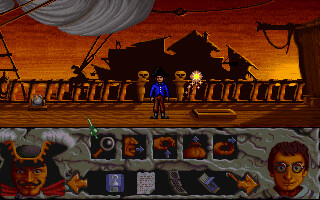This is a detailed screenshot from the animated video game "Hook," capturing an intense scene aboard a pirate ship. At the center of the ship stands a pirate wearing a blue shirt, brown pants, and a black hat, gazing forward with a determined expression. Flanking him are two ominous skulls, adding to the ship's eerie ambiance. To the front left, we see Captain Hook himself, distinguished by his black hat trimmed in yellow, a striking mustache, and a red bow around his head. On the right, an animated man wearing glasses adds to the eclectic crew. In the background, another ship looms, suggesting an unfolding maritime adventure. This vivid scene encapsulates the adventurous spirit of the game.